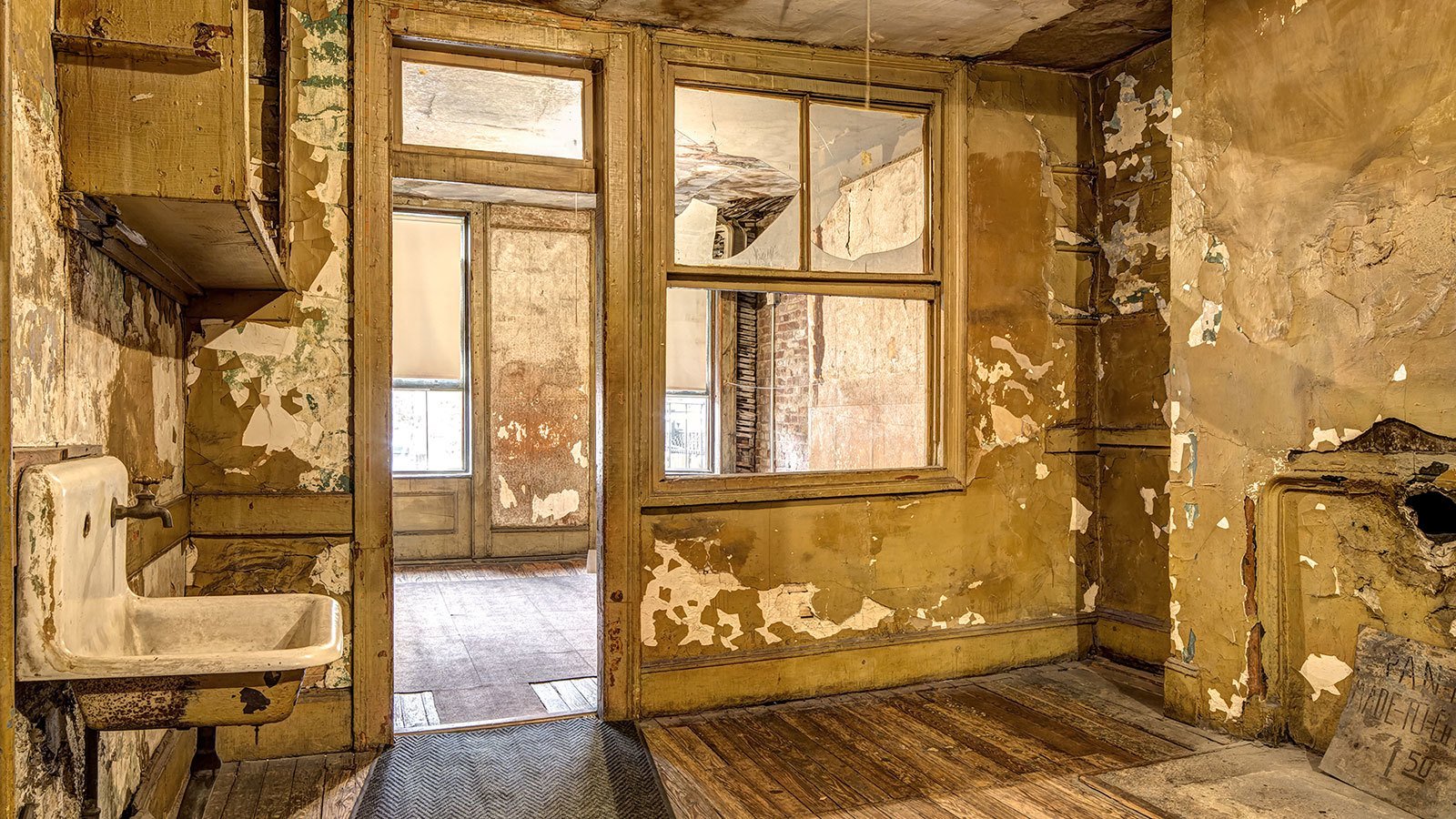The image depicts an extremely run-down room, possibly a bathroom, situated inside an old, abandoned building. This room lacks a door in its frame but features a window above it and another to the right, which allows a view into an adjacent room. The walls, primarily wooden, are severely tattered, with extensive peeling paint and remnants of wallpaper. Numerous holes punctuate the walls, and light spills in from the front room's windows, which have shades pulled up a third of the way.

On the left-hand side of the room sits a dilapidated sink with an antique faucet, missing its drain pipe. Above it, a weathered cabinet hangs precariously. The sink itself shows signs of severe wear, with blackened patches and areas of rust. A cord hangs from the ceiling, possibly for a light fixture.

To the right, the wall features an indent and a small, filthy sign on the ground, which is largely illegible except for the text "$1.50" at the bottom, perhaps suggesting a past commercial use of the space. The flooring is a dark, unfinished wood that adds to the room's overall neglected appearance. The scene captures an environment of decay and abandonment, with every element contributing to its derelict state.